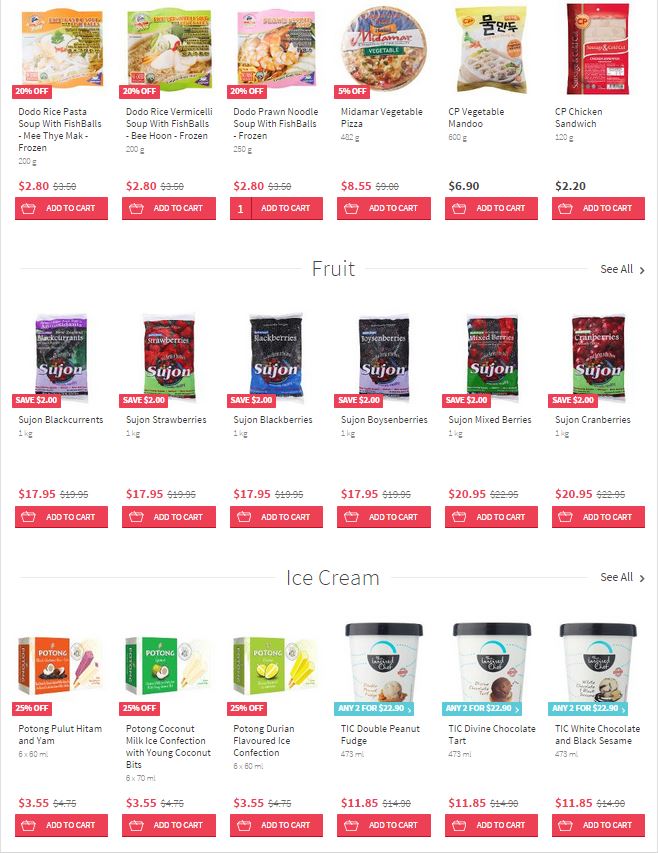The image displays a landing page for a grocery store, structured with three rows of six products each, totaling 18 visible items. 

- **First Row**: A variety of pasta products and quick meals dominate this row. The first three items, mostly instant ramen, are priced at $2.80 each. Following these, the fourth item is a Vegetable Pizza priced at $8.55. The fifth product, a Vegetable Mandu, is $6.90. The row concludes with a Chicken Sandwich priced at $2.20. Each product features an "Add to Cart" button along with its respective price displayed prominently at the bottom.

- **Second Row**: This row is dedicated entirely to fruit products from the brand Sujon. The sequence begins with Sujon Blackcurrants, followed by Sujon Strawberries, Sujon Blackberries, and Sujon Boysenberries, all priced at $17.95 each. The final two items in this row are Sujon Mixed Berries and Sujon Cranberries, both available for $20.95. 

- **Third Row**: Focused on ice cream, this row showcases items from two brands. The first three items, each priced at $3.55, are from the brand Poton. The last three items are from TIC and include TIC Double Peanut Fudge, TIC Divine Chocolate Tart, and TIC White Chocolate and Black Sesame, each priced at $11.85.

Each product is clearly labeled with its name and price, emphasizing the visual organization and ease of shopping on this grocery store's landing page.